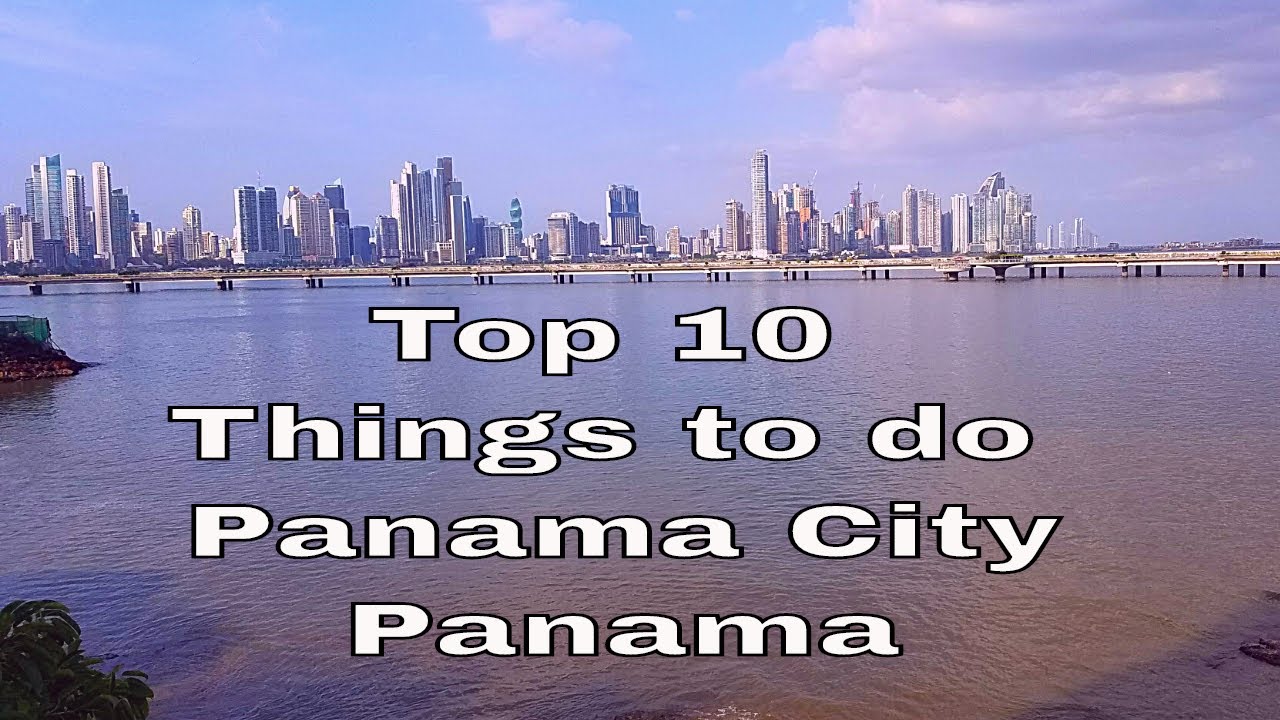The image depicts a stunning panorama of Panama City, Panama. On the left side of the sky, there is a brilliant blue hue that gradually transitions into a more cloudy sky with shades of purple towards the right. Dominating the scene below is a city skyline filled with towering skyscrapers that stretch across the entire width of the image, except for a small gap on the right. Below the skyline, a prominent bridge spans from left to right above a large body of water. On the left side, a small island is visible, albeit somewhat indistinct. In the bottom left corner of the image, part of a tree can be seen, while the lower portion of the image reveals a shadow cast across the water. Centrally positioned in white text, the image is overlaid with the title: "Top Ten Things to Do, Panama City, Panama." The image is devoid of any people, showcasing purely the urban and natural landscape.